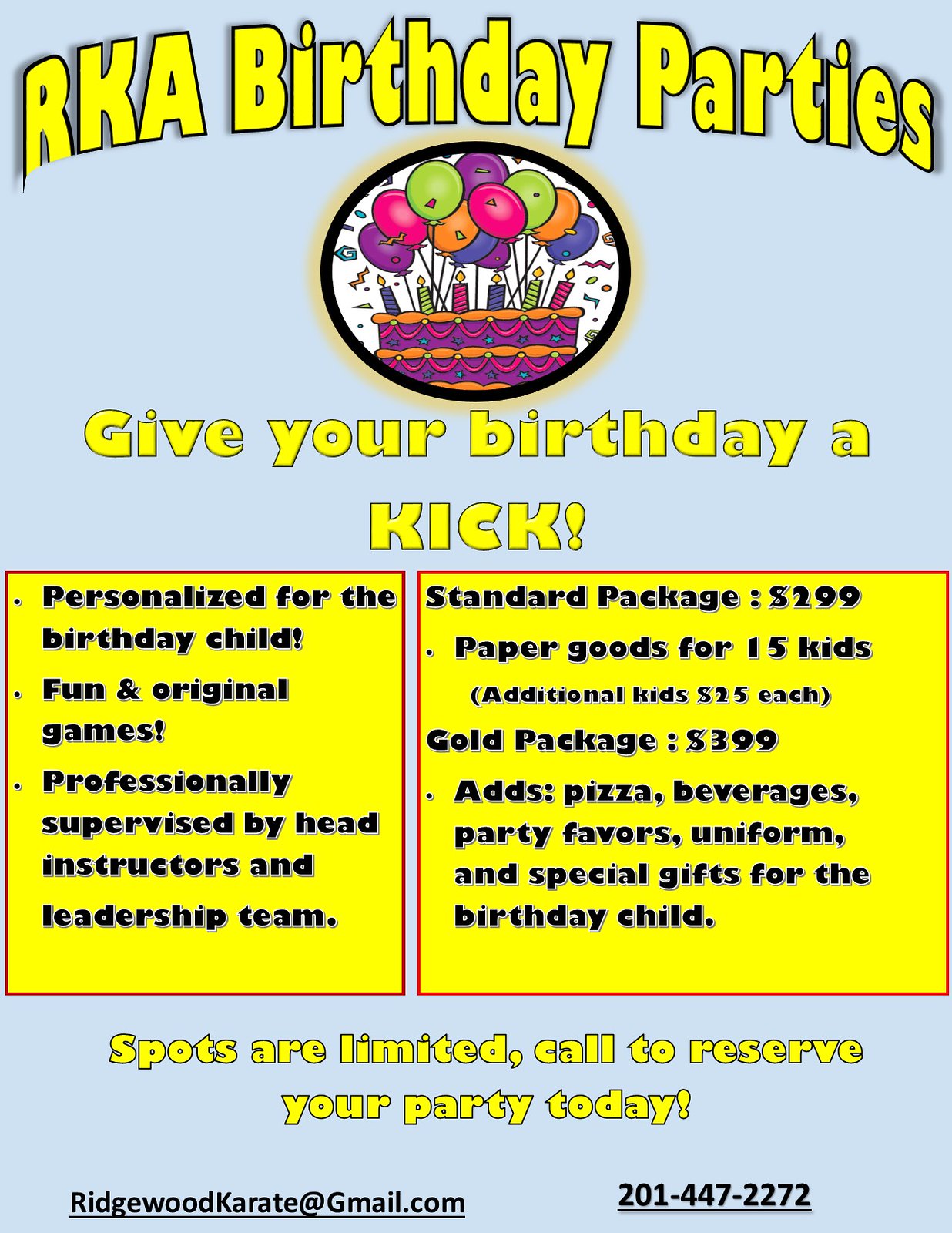This advertisement for RKA Birthday Parties features a vibrant blue background with bold yellow text across the top that reads, "RKA Birthday Parties." Beneath the title is a colorful, digitally produced image of a birthday cake adorned with candles, surrounded by bright balloons in shades of orange, purple, pink, and green. The midsection of the ad declares, "Give Your Birthday a Kick," also in yellow print. Further down, black text on yellow backgrounds provide detailed information about the party packages offered. The left column details that the parties are personalized for the birthday child, include fun and original games, and are professionally supervised by head instructors and leadership team. The right column outlines the packages: the standard package for $299, which includes paper goods for 15 kids, with additional kids at $25 each, and the gold package for $399, which adds pizza, beverages, party favors, uniforms, and special gifts for the birthday child. The advertisement stresses that spots are limited and includes contact information at the bottom: RidgewoodKarateGmail.com and a phone number, 201-447-2272, encouraging immediate booking.